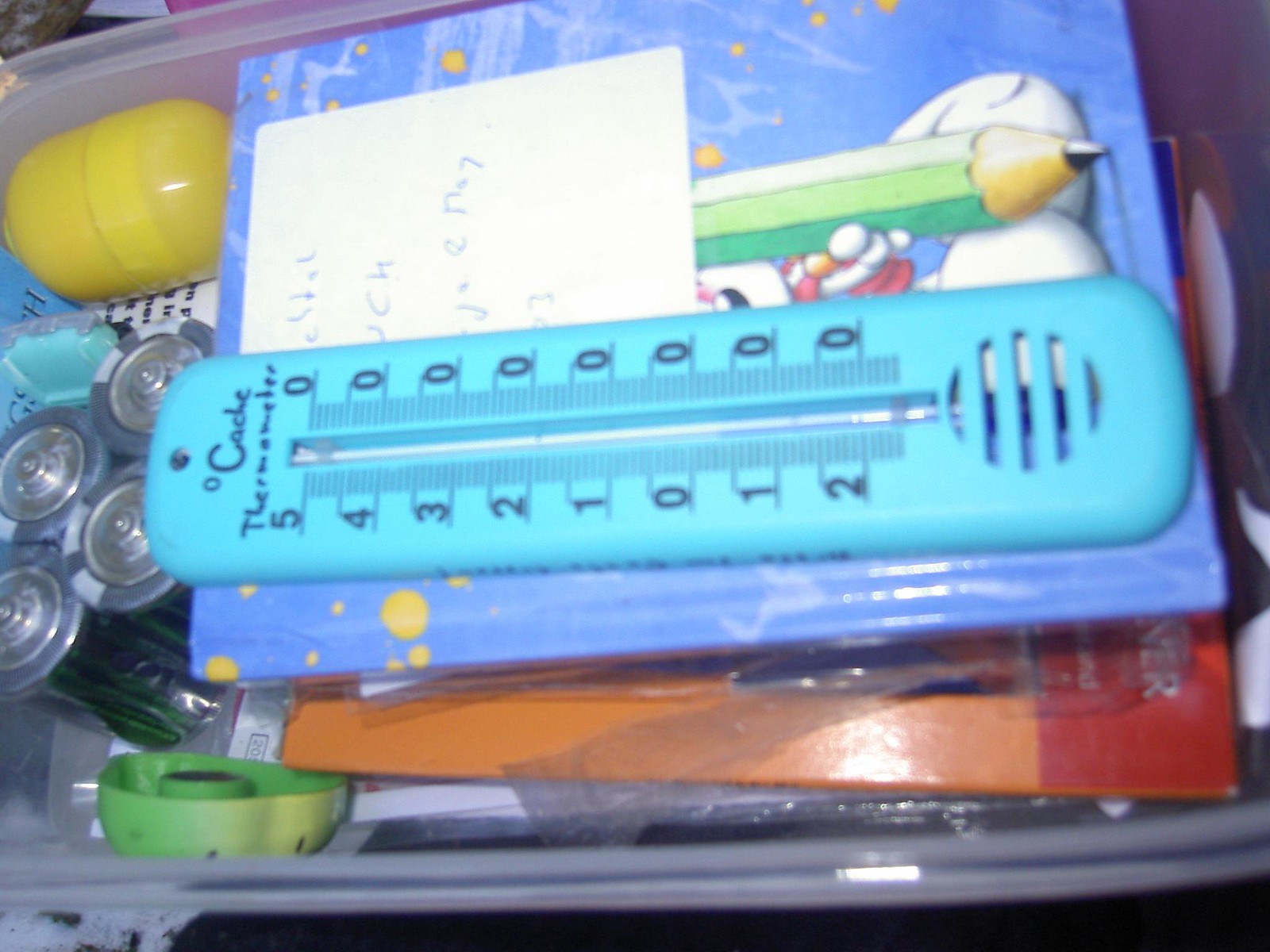This photograph showcases the neatly arranged contents of a translucent white plastic storage box, featuring an assortment of household and stationery items. Among the items, a notebook is prominently visible, marked with a post-it note inscribed in blue ink. Adjacent to the notebook lies a wall-mounted thermometer, designed in blue plastic with black print, indicating temperature in degrees Celsius. The box also contains a couple of D-size batteries and a small yellow plastic capsule container. A green plastic object, outfitted with a button magnet on the back, is also part of the collection. Additionally, a cardboard box that appears to store pencils completes the diverse assortment within the container.